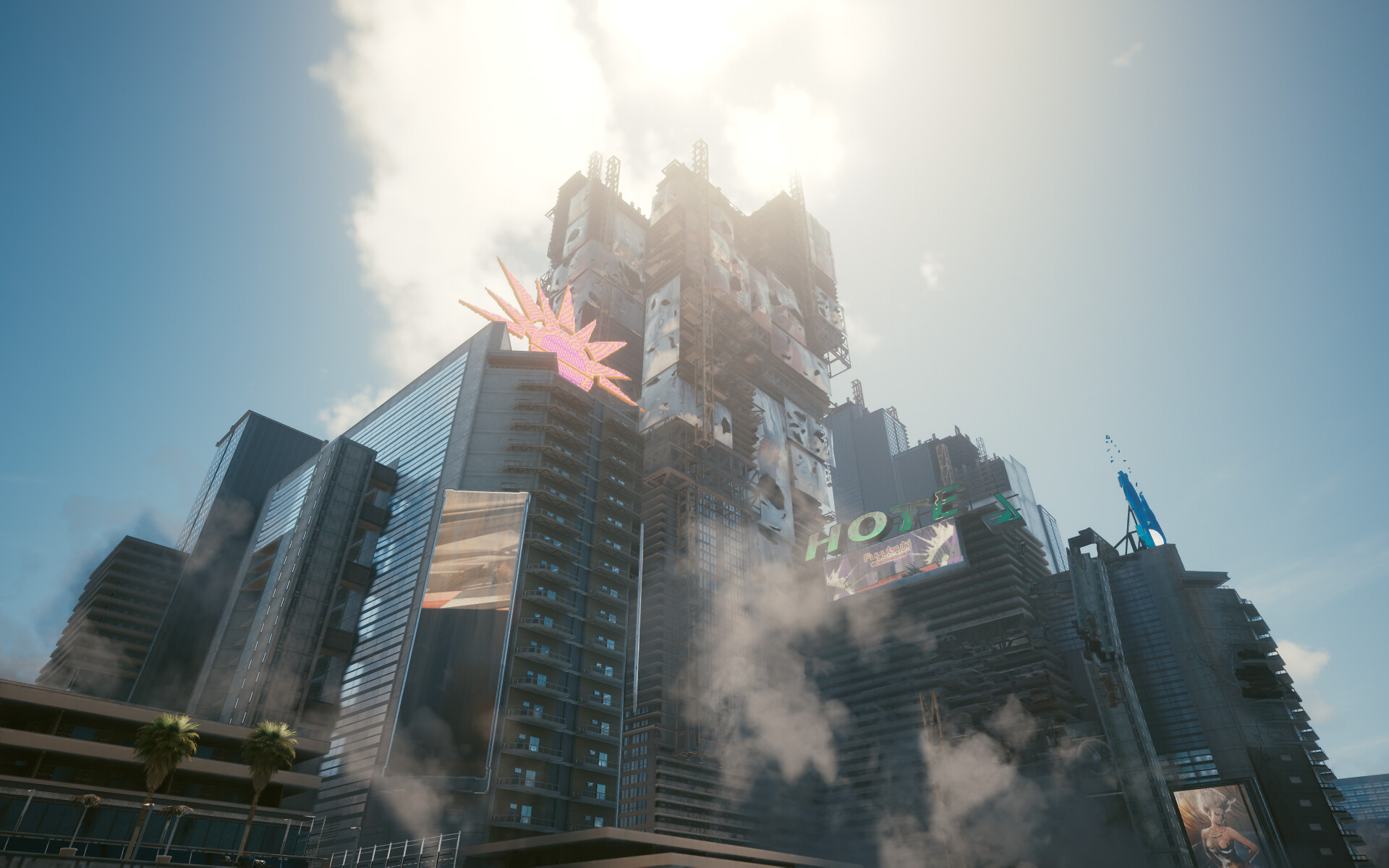A towering, dilapidated structure dominates the scene with an unmistakable post-apocalyptic aura. The most striking feature is a partially lit sign that once read "HOTEL," but now displays "HOTE" in faded green letters, the 'L' having fallen off. Below it, a small, weary billboard clings to the façade. The building is an immense aggregation of what seems like multiple skyscrapers haphazardly fused together, featuring an assortment of balconies that likely served as condos. Above these residential sections, the structure transitions into an industrial wasteland, with crumbling parts belching faint plumes of smoke. The backdrop consists of a clear blue sky adorned with scattered, white clouds, offering a stark contrast to the grim decay below. Atop one of the decrepit towers, a prominent red star emblem stands, possibly hinting at the building's storied past.